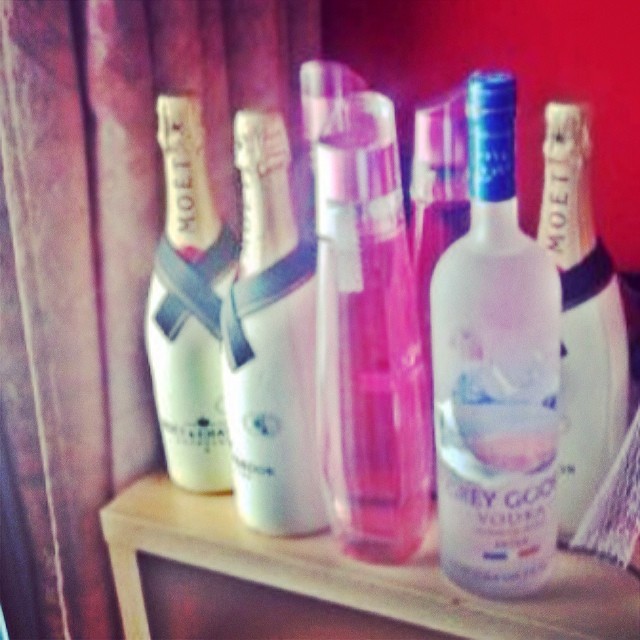The photograph features an assortment of bottles of alcohol displayed on a light tan wooden cabinet against a deep red wall backdrop, accompanied by greyish curtains to the left. The image, possibly filtered to appear older, exhibits a reddish hue with slightly faded, blurry colors. 

Prominently positioned are three white bottles adorned with gold tops and dark ties across their fronts, identified as Moet champagne, which is unmistakable due to the "M-O-E-T" text on their necks. Among them are three clear bottles containing a pinkish liquid, creating a striking contrast. In front of this arrangement, two unopened white bottles feature blue bands under their necks. 

Additionally, a clear bottle of Grey Goose Vodka with a royal blue top sits at the bottom right corner of the cabinet. The overall composition suggests a celebration or display, with the varied bottle shapes, sizes, and contents providing a visually appealing assortment of alcoholic beverages.